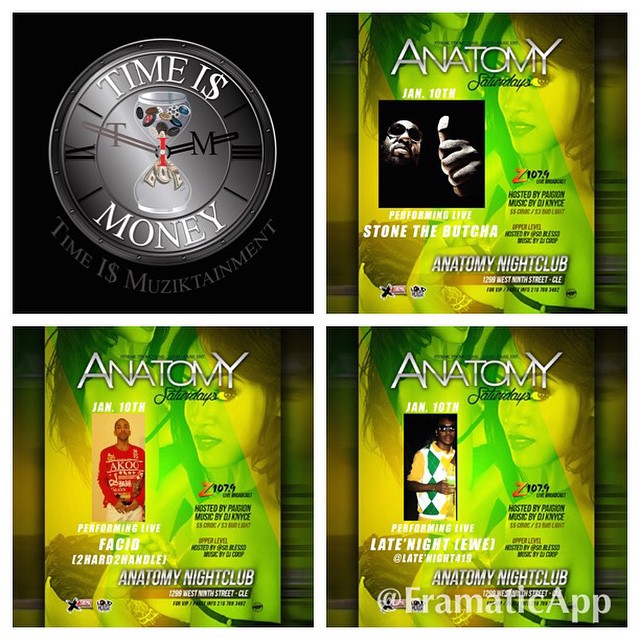The image features a green-themed background with a prominent timepiece displaying the phrase "Time is Money." The watch, or timepiece, has uniquely labeled hands marked with "P" and "M." Surrounding the watch are three distinct yet similar advertisements promoting different anatomy clubs, each showcasing a collection of books by various artists. One of these ads is titled "Late Night" and is attributed to the artist Chromatic Black. Each advertisement features an identical dancer woman with expressive, wide eyes, who appears in the green-background setting. Although each ad changes the featured dancer, the overall theme and design remain consistent, highlighting the notion that time is an essential factor in the pursuit of art and knowledge.